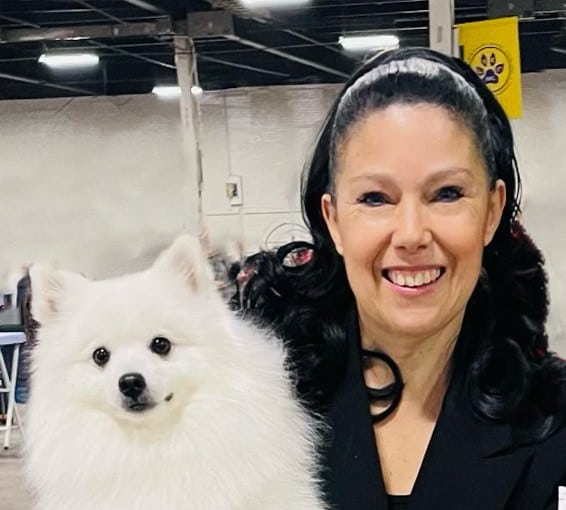In the image, a middle-aged woman, likely in her 40s or 50s, is smiling warmly at the camera. She has long, curly black hair accented with a white headband, and a touch of grey at her temples. Her hair cascades over her shoulders. She's wearing thick black eyeliner and visibly has some wrinkles around her eyes. Her big smile reveals the top of her teeth distinctively. She is dressed in a formal black jacket with a low neckline, possibly layered over a black undershirt.

To her left, she is holding a small, very fuzzy Pomeranian dog. The dog is predominantly white with black eyes, a black nose, and a little black mouth. Behind the woman, near the top right corner of the frame, there's a white pole with a yellow flag featuring a paw print, hinting at a possible dog competition setting. The background appears to be within a warehouse-like environment, with a white table and blue chair visible to the back left of the dog, under a dark ceiling adorned with hanging white lights.